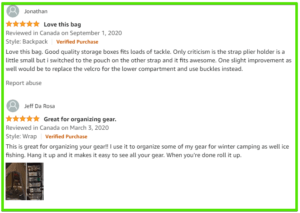**Detailed Caption:**

The image is a screenshot displaying two Amazon product reviews, outlined by a bright green horizontal rectangle. 

**Review 1 by Jonathan:**
Jonathan's review is titled "Love This Bag" and he gave it a 5-star rating. The review, marked as a verified purchase, was written in Canada on September 1, 2020, under the "style backpack" category. Jonathan praises the bag for its good quality and ample storage, ideal for holding a large amount of tackle. However, he notes that the strap plier holder is a bit small, although he fixed this by using the pouch on the alternate strap, which works perfectly. He also suggests an improvement - replacing the Velcro on the lower compartment with buckles for better functionality. The review ends with an option to "Report abuse."

**Review 2 by Jeff DeRosa:**
Jeff DeRosa's review, also rated 5 stars, is titled "Great for Organizing Gear." His review, another verified purchase, was posted in Canada on March 3, 2020, under the "style wrap" category. Jeff speaks highly of the product’s capability to organize gear, particularly useful for winter camping and ice fishing. He appreciates the convenience of hanging it up to easily access his gear, and notes that it can be rolled up neatly when finished. Additionally, Jeff's review includes some photos showcasing the product in use.